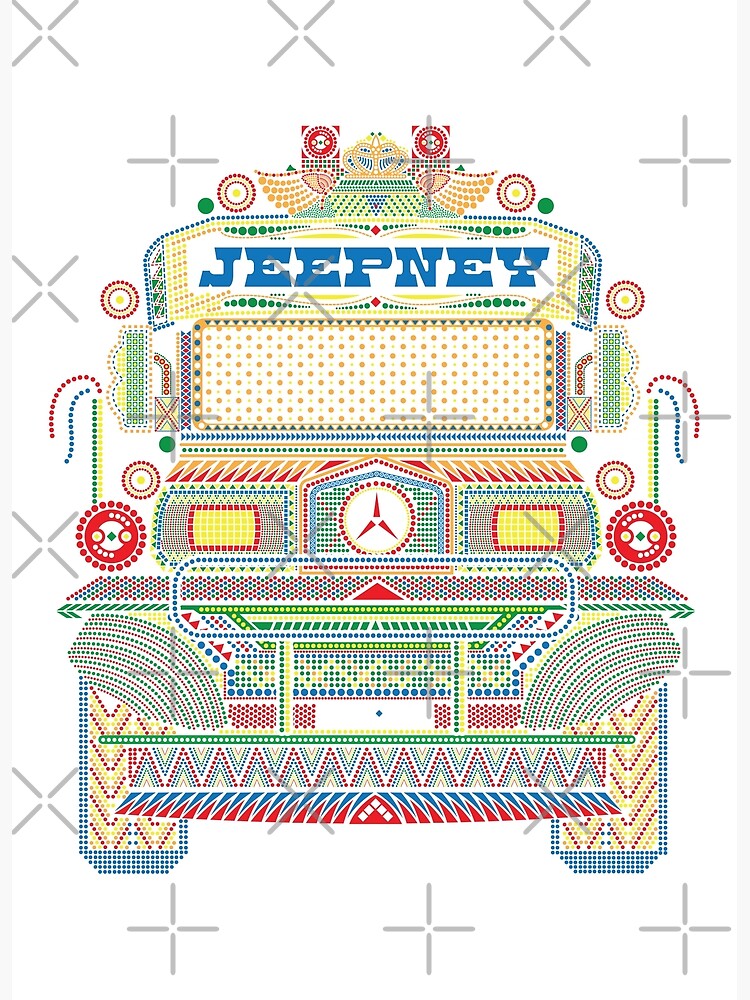In this captivating artwork, the background is white with a semi-transparent overlay of black and gray X's and plus signs, creating a watermark effect that doesn't obscure the main image. The central focus is a colorful depiction of a vehicle, presumably a Jeepney, formed entirely from an array of vibrant dots in various hues including red, blue, yellow, gold, and green, reminiscent of a lively carnival atmosphere. Intricately detailed, the vehicle's windshield features golden dots on a white background, and a white emblem with three slender triangles, possibly echoing a Mercedes logo, is situated where a traditional carmaker's logo would be. The Jeepney title is prominently displayed in blue across the top of the windshield. Each component of the vehicle, from its tires and headlights to the mirrors and grille, is crafted from these colorful dots, showcasing a playful and whimsical design.